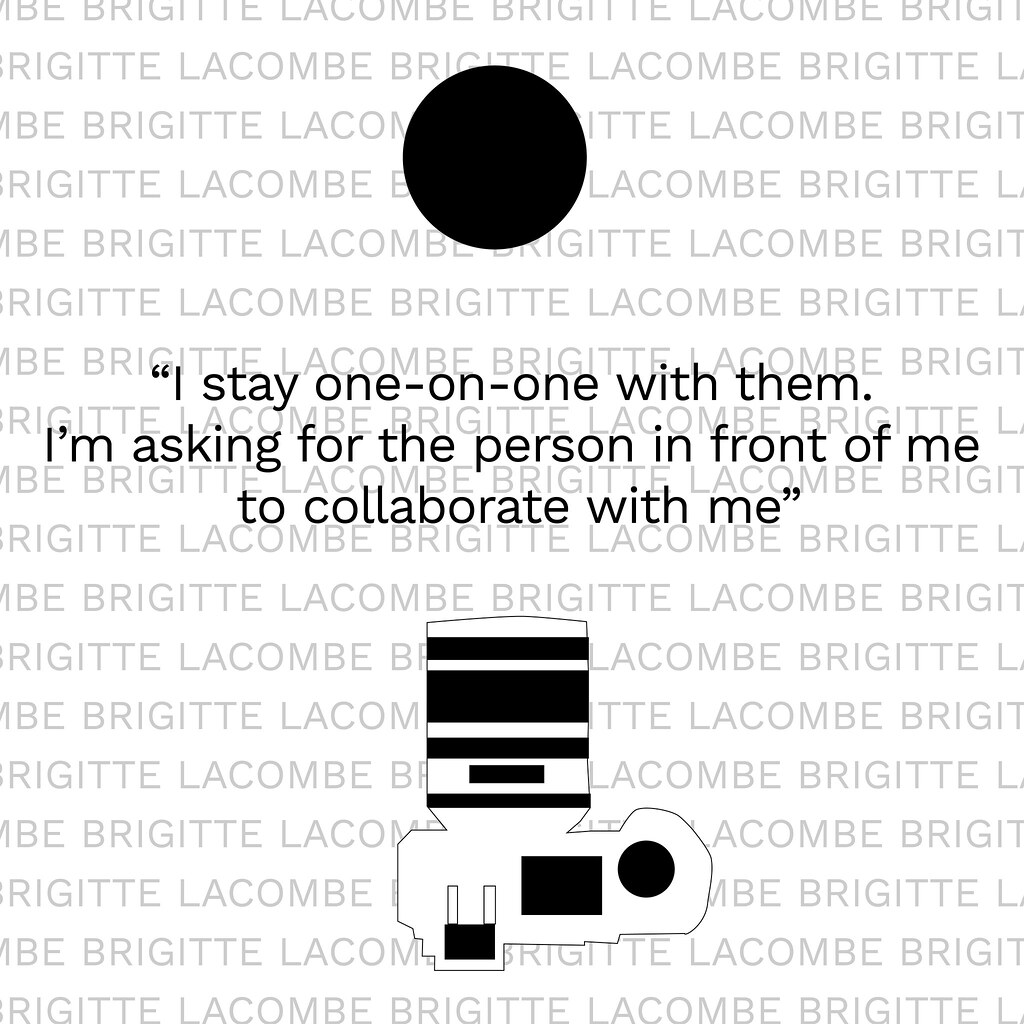The image features a white background densely covered with the text "Brigitte Lacombe" repeated in light gray, creating a subtle, offset, and parallel pattern. At the top of the image, there is a prominent gray circle. Below this circle, centered in dark gray letters, is a quote: "I stay one-on-one with them. I'm asking for the person in front of me to collaborate with me." Underneath the quote, there is a black and white schematic drawing that appears complex and somewhat ambiguous. The drawing includes a cylindrical shape on top, resembling either a water tank or a component of a vehicle engine, and an irregular rectangular base with various protrusions. Scattered across the schematic are gray bars and a circle, adding to the technical aesthetic of the design.